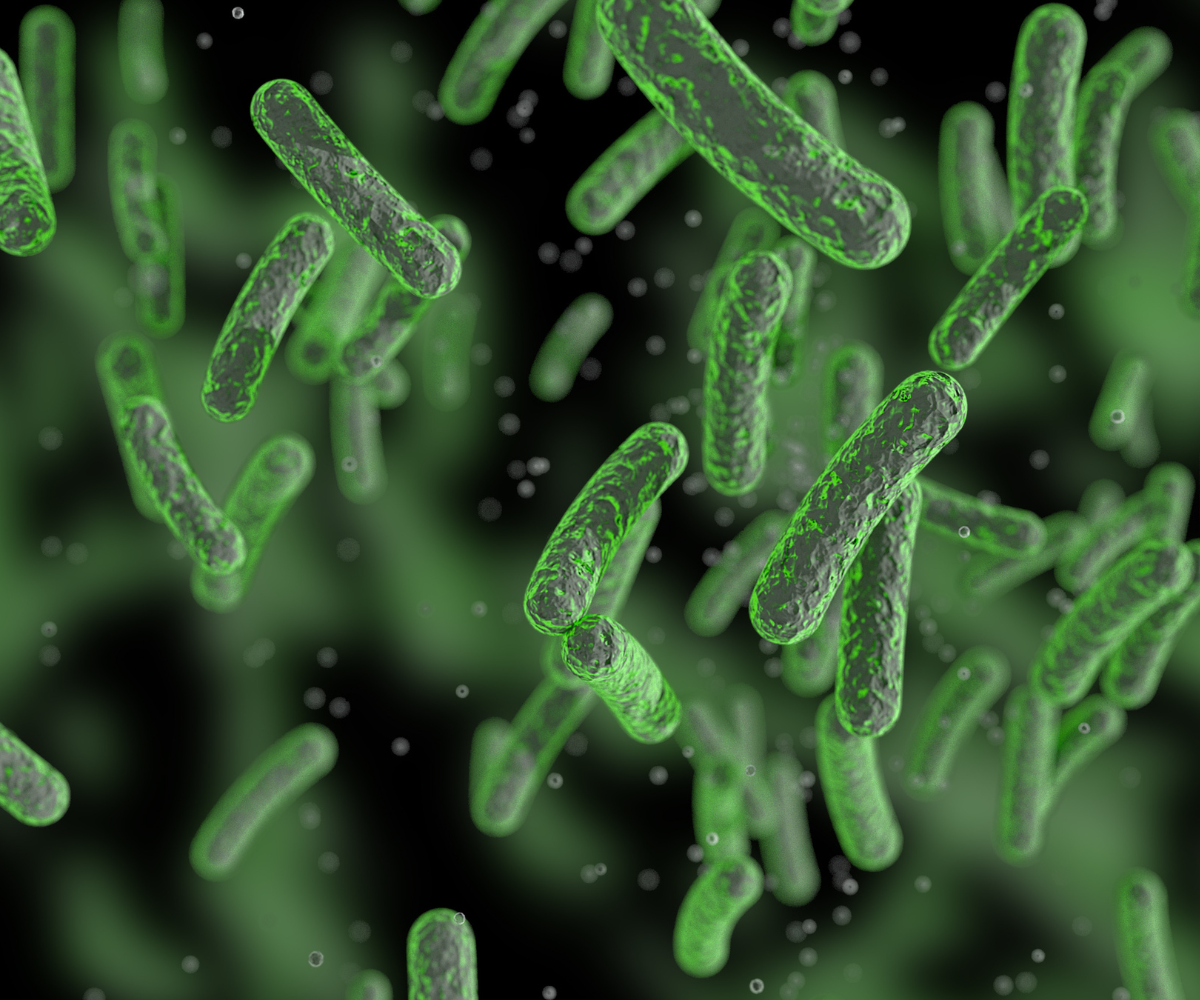The image is an AI-generated visualization of microscopic bacteria or amoeba-like cells, vividly resembling lime-green, pill-shaped or hot dog-shaped rods. These cellular forms are dispersed throughout the image, with some prominently focused in the foreground while others remain blurred in the background. The scene is strikingly monochromatic, dominated by neon green hues contrasted against patches of deep black and gray. The background is a blurred mix of these colors, with occasional white bubbles adding subtle depth. The overall effect is a highly detailed, bright, and surreal representation of microorganisms suspended in a dark, indistinct environment.